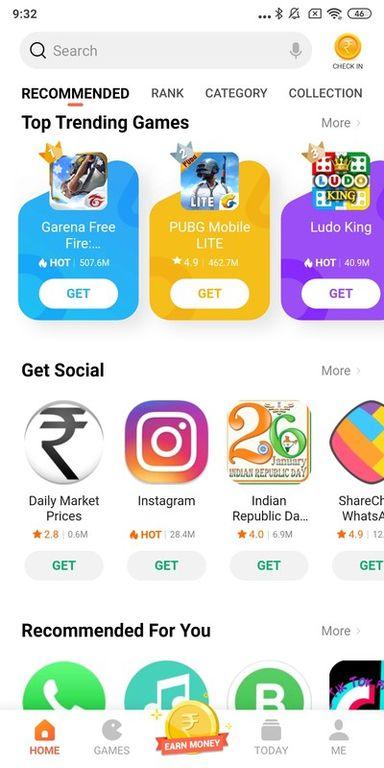This image appears to be a cropped screen capture of an older Android phone, likely experiencing heavy artifacting from multiple shares or poor image compression. The interface showcases a predominantly white background with a black clock display reading "9:32" at the top. Adjacent to the clock are the battery and Wi-Fi icons located on the far left. Directly below this, a gray search bar is present, accompanied by a yellow-gold "Check In" button on its right.

Further down, a navigation section marked "Recommended," "Rank," "Category," and "Collection" is visible, with "Recommended" being highlighted in bold and underlined by a small red line. The screen displays a list under "Top Trending Games," featuring titles like "PUBG Mobile Lite," "Arena Free Fire," and "Ludo King," each adorned with multicolored icons and white "Get" buttons.

The "Get Social" section follows, suggesting side-to-side scrolling capability. The icons here include "Daily Market Prices," "Instagram," "Indian Republic," and partially visible "Share something" and "WhatsApp." Finally, a "Recommended for You" segment lists basic app icons, such as a phone symbol, a music note, and another with a bee inside a green circle.